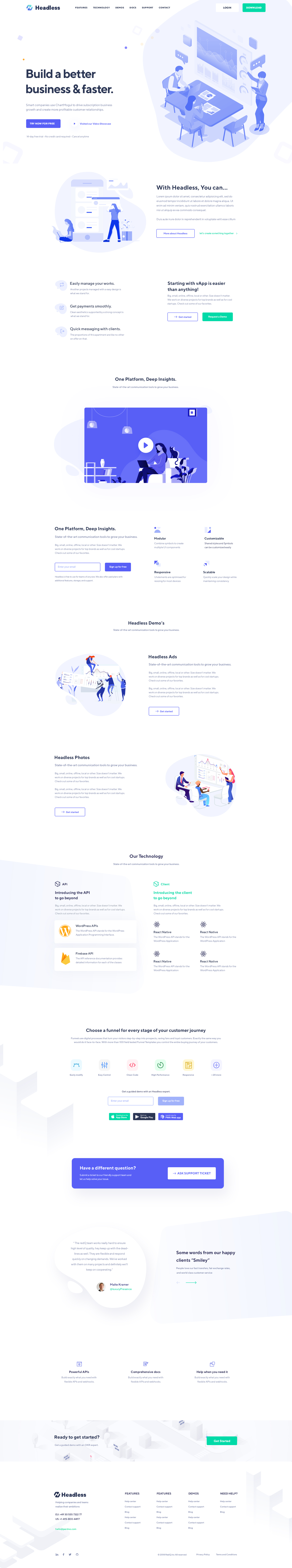The image depicts a webpage, viewed from a distance, with elements too small to discern in detail. In the upper left corner, there is a bluish-colored logo followed by black text indicating the name of the brand or company. To the right of the logo and text, there are black navigation tabs for different categories that allow users to explore specific sections of the site. In the upper right corner, there are login and signup buttons, distinguished by green and white colors respectively.

Beneath the top bar, there's an image of an office scenario where someone appears to be giving a presentation on a board while two individuals are working at a desk. Overlaid on this image is the text "Build a Better Business Faster."

Following this, more informational content is provided. Below this section, there's a video thumbnail featuring a purple and white color scheme, inviting users to watch the related video. Further down, additional information is presented along with a section where users can sign up with their email address. Lastly, the bottom of the page contains more informational content, completing the comprehensive overview of the webpage.